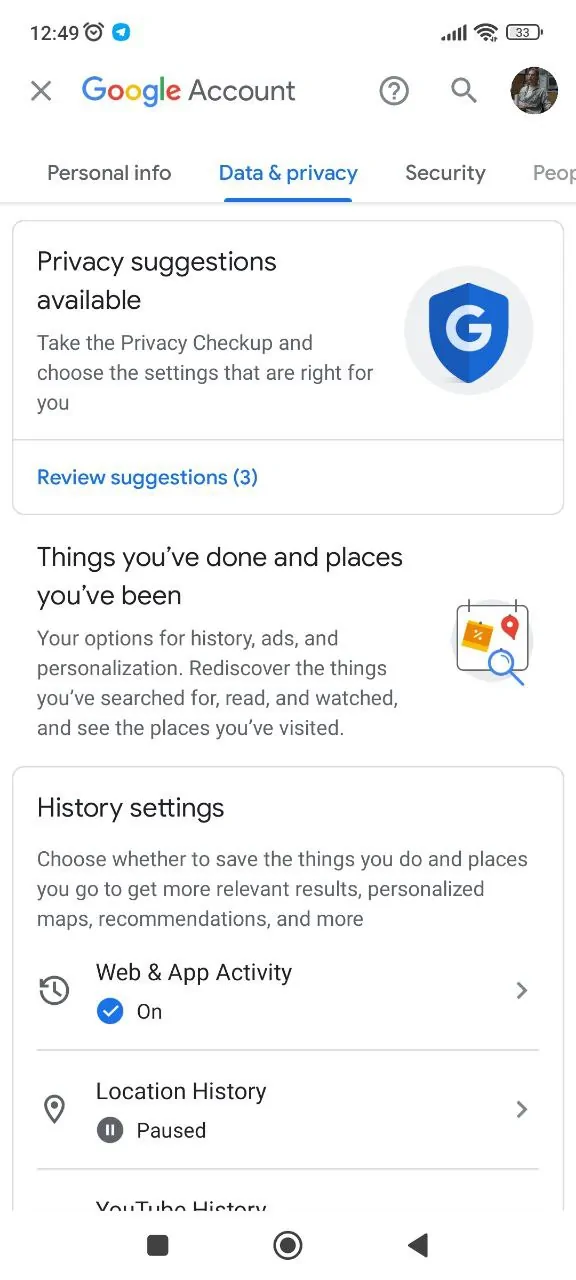The image is a screenshot of a Google Account page taken on a device with a 33% battery level, indicated at the top right of the interface. The timestamp shows 12:49. At the top of the image, the Google logo is prominently displayed next to the word "Account" in black text. There are several tabs available: "Personal info," "Data and privacy," and "Security," with the "Data and privacy" tab selected and highlighted in blue.

Directly below the tabs, there is a boxed section with a white background labeled "Privacy suggestions available." The text below this label invites the user to "Take the privacy checkup and choose the settings that are right for you." To the right of this message is a blue shield icon featuring a white "G," accompanied by the text "Review suggestions (3)."

Further down, there's another section titled "Things you've done and places you've been," which outlines options related to history, ads personalization, and rediscovering past searches, reads, watches, and visits. Under this heading is a black text box labeled "History settings," guiding the user to "Choose whether to save the things you do and places you go to get more relevant results, personalized maps, recommendations and more."

Within the "History settings" box, three specific activities are mentioned: "Web & App Activity," which is turned on, "Location History," which is paused, and "YouTube History." Unfortunately, the image cuts off at this point, preventing further readability. At the very bottom of the image, three buttons are visible: a gray square, a gray circle, and a gray triangle pointing to the left.